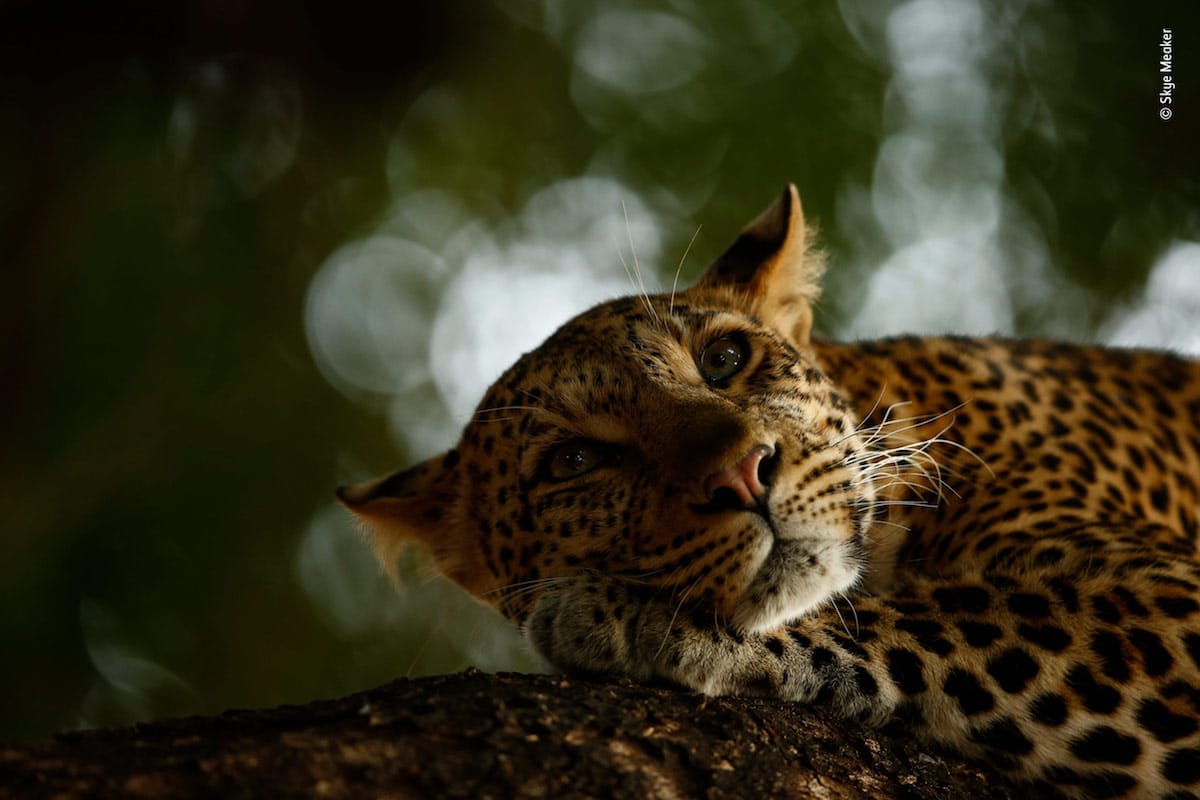This close-up color photograph features a resting leopard, its light brown fur marked with distinctive black spots. The leopard's head reclines on its left paw, which is draped over a black and light brown tree trunk. Its pink nose and white whiskers stand out prominently, while its ears, covered in gold fur, are adorned with tufts of hair. The leopard's eyes are open, gazing out into the distance, giving the image a serene yet attentive quality. Only part of its body is visible, extending to the right about halfway down the frame, with the rest obscured. The background is a blurred mixture of dark green foliage and out-of-focus white circles, suggesting sunlight filtering through the trees. At the top right corner, a watermark reads "copyright Skye Meaker" in white text. The entire composition emphasizes the leopard in repose while hinting at its natural habitat beyond the lens.